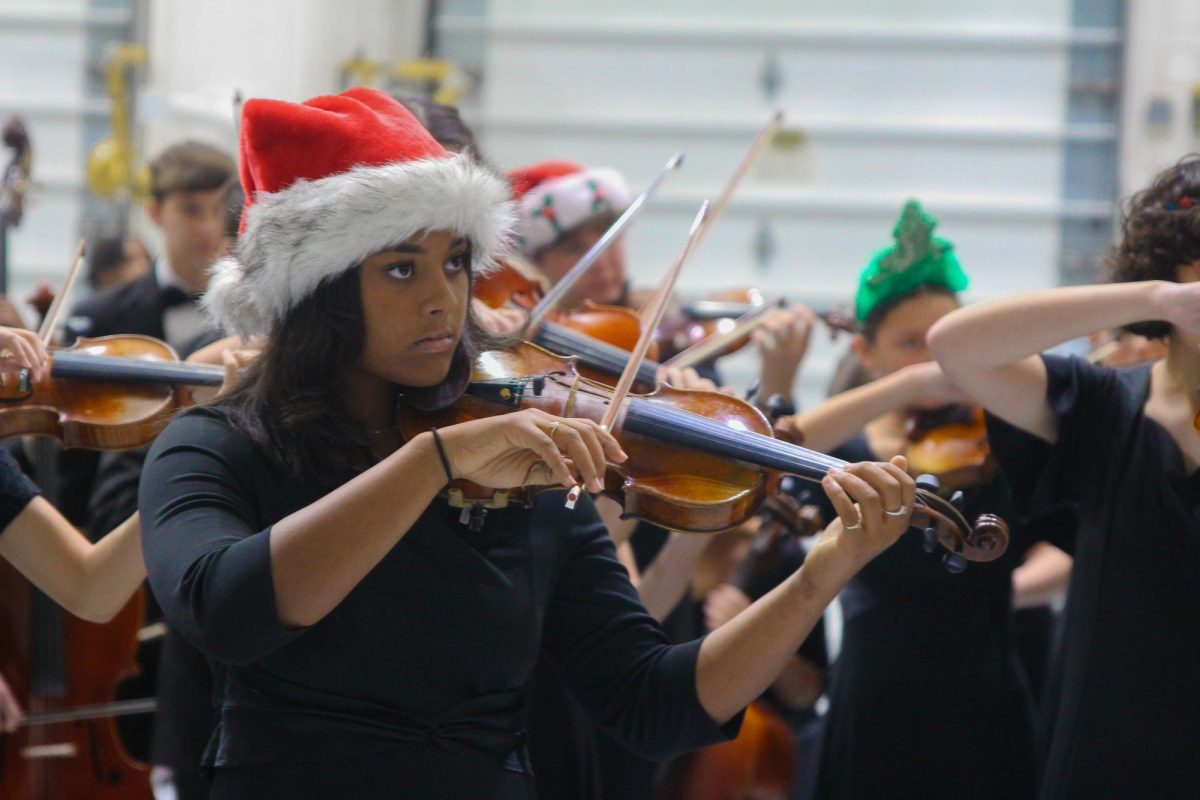The photograph depicts a group of students performing indoors as part of a choir or band ensemble, primarily focusing on string instruments like violins. The central figure is a brown-skinned girl with dark brown hair, wearing a traditional Santa hat with white, fluffy trim and red velvet. She is dressed in a black shirt with three-quarter length sleeves, playing a wooden violin, holding the bow in her right hand while the violin rests under her chin. Surrounding her are other students similarly dressed in black outfits—ranging from t-shirts to long-sleeve shirts and dresses—all diligently playing their violins. In the background, one student wears a distinctive green hat resembling a Christmas tree, another sports a Santa hat adorned with green holly leaves, and a young boy also in a Santa hat. The backdrop features light gray, industrial-style metal doors, contributing to a subtle, utilitarian ambiance, with blurred figures and instruments enhancing the focus on the main violinist in front.